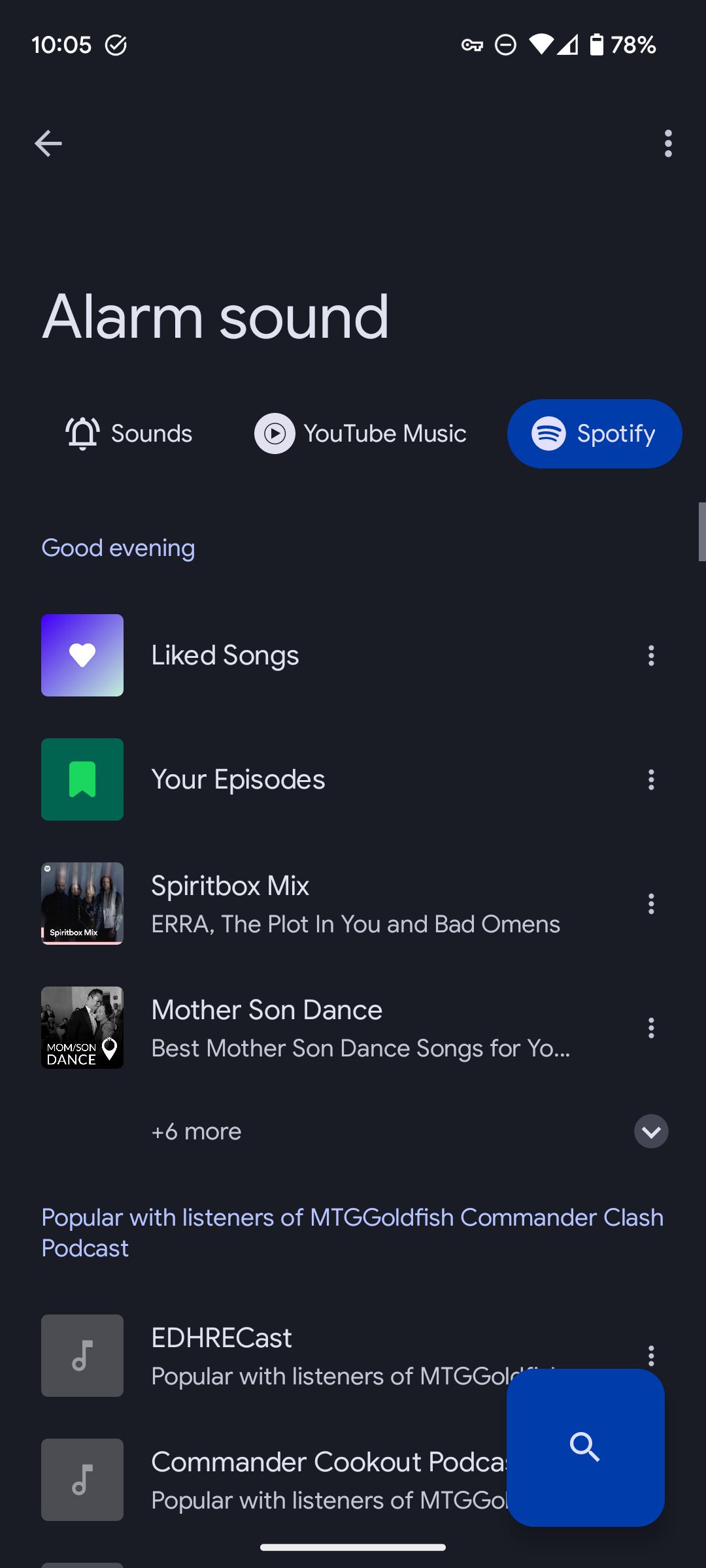The image is a portrait-oriented screenshot from a cell phone, set against a completely black background, creating a stark, visually distinct single-column layout. In the upper left corner, the time is displayed as 10:05, accompanied by a check mark. The upper right corner shows the battery status at 78%.

In the subsequent row, there is a back arrow on the left and a menu button with three vertical dots on the right. Below this, in a very large font, the words "Alarm Sound" are prominently displayed. The following row features several icons: a bell icon, a sound icon, the YouTube logo, the YouTube Music logo, and a highlighted blue button for Spotify, indicating the current selection.

The screen appears to be the interface for choosing an alarm sound, and it greets the user with "Good evening." Beneath this greeting, there are four rows, each containing an image on the left and corresponding titles and descriptions:

1. The first row features an image of a heart against a light blue background with "Liked Songs" as the title.
2. The second row displays a light green bookmark on a dark green background, labeled "Your Episodes."
3. The third row contains a blurry image and is titled "Spirit Box Mix, ERA, The Plot In You, and Bad Omens."
4. The fourth row shows an image of a man and a woman with the title "Mother Son Dance, Best Mother Son Dance Songs For You" followed by a note indicating there are "+6 more" items.

At the bottom, there is additional information stating, "Popular with listeners of MTGGoldfish, Commander Clash Podcast, EDHRECast, and Commander Cookout."